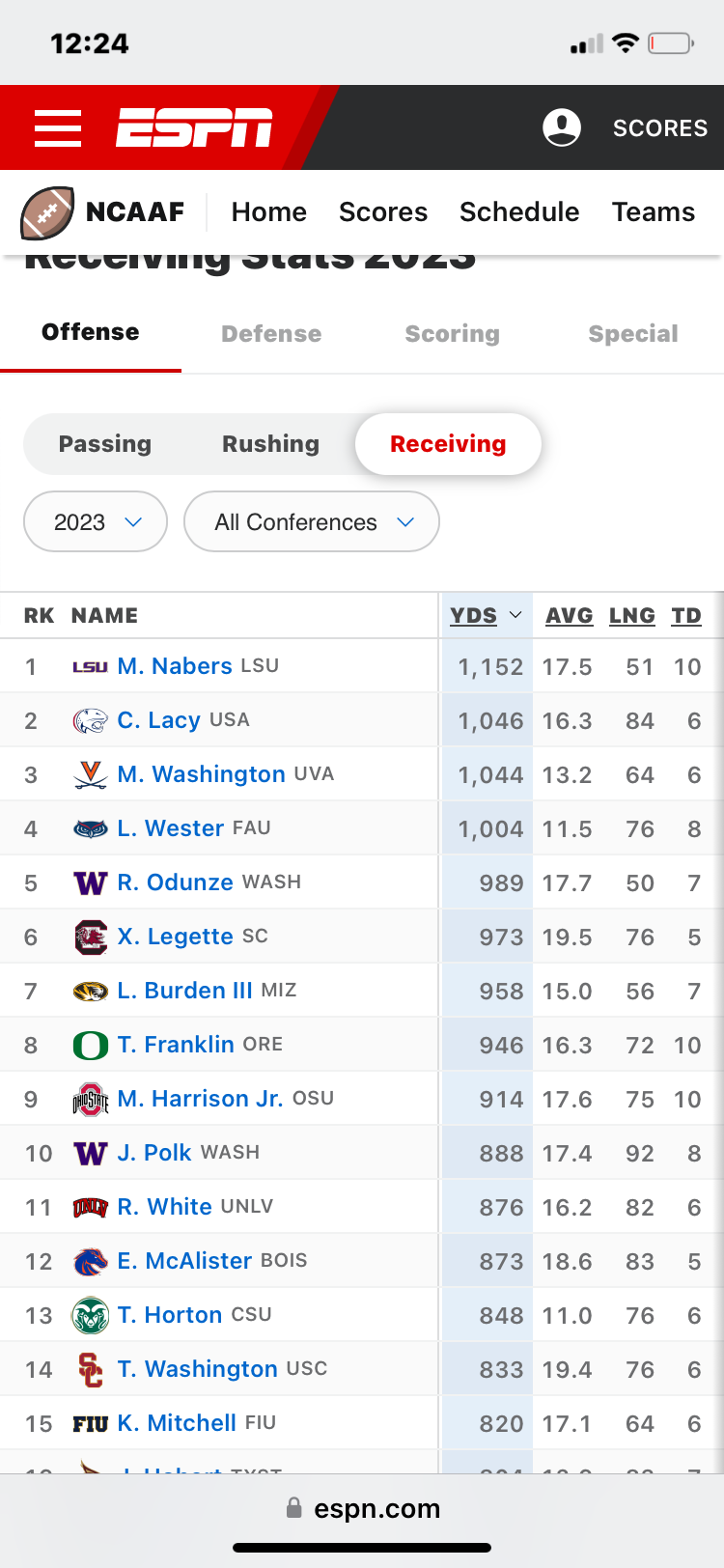This mobile screenshot of an ESPN website captures several details carefully arranged on the screen. In the top left corner, the time is displayed as 12:24. The top right corner features a Wi-Fi symbol and a battery icon that shows only a tiny red sliver, indicating the phone is about to run out of battery.

The banner just below the header sports a gradient design with red on the left and black on the right. This banner holds the ESPN logo, a profile picture icon, and a "Scores" link on the far right. Directly beneath this is a section focused on NCAA Football, labeled as "NCAAF," which includes four navigational tabs: Home, Scores, Schedule, and Teams.

The main content area is divided into sections titled Offense, Defense, Scoring, and Special Teams, with "Offense" underlined by a red line to indicate it as the selected category. A secondary menu beneath this offers options for Passing, Rushing, and Receiving, with "Receiving" highlighted in red text. Two dropdown menus follow, allowing users to filter by "2023" and "All Conferences."

At the core of the page is a table that ranks 15 players according to various performance metrics, including columns for Rank, Name, Yards (YDS), Average (AVG), Longest (LNG), and Touchdowns (TD). The players' names are displayed in blue text, accompanied by their respective team icons on the left.